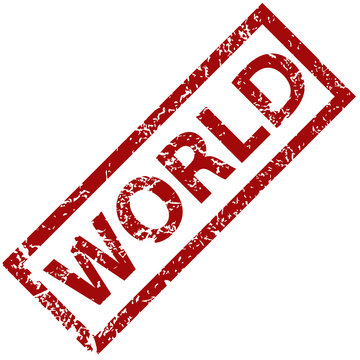The image is a simple, digitally-produced illustration on a pure white background. It features the word "WORLD," spelled W-O-R-L-D in bold, all-capital red letters. The letters are on an upward-right angle, running from the lower left-hand corner to the upper right-hand corner. Surrounding the word is a rectangular red border of the same thickness as the letters. Both the letters and the border have a distressed, faded look, with veins or squiggles of white running through the red, giving them a crackled appearance. This creates a textured effect within the uniform color scheme of red and white.